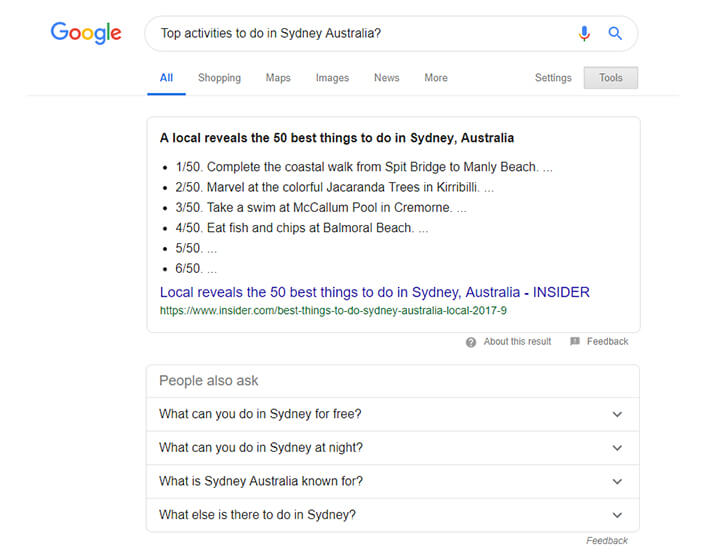The image shows a Google search query typed in black within the search bar, reading "top activities to do in Sydney, Australia." The search results begin just below the search bar. The first link displayed states, "A local reveals the 50 best things to do in Sydney, Australia," with a snippet listing the top six activities. 

1. (1/50) Complete the coastal walk from Spit Bridge to Manly Bridge.
2. (2/50) Marvel at the colorful Jacaranda trees in Kirribilli.
3. (3/50) Take a swim at MacCallum Pool in Cremorne.
4. (4/50) Eat fish and chips at Balmoral Beach.
5. (5/50) [Not visible in the image]
6. (6/50) [Not visible in the image]

Beneath this, the summary repeats, "A local reveals the 50 best things to do in Sydney, Australia," written in blue. The associated URL, displayed in green, reads "insider.com/best-things-to-do-sydney-australia-local-2017-9." 

At the bottom of the search results, Google suggests additional related questions under the "People also ask" section:

- What can you do in Sydney for free?
- What can you do in Sydney at night?
- What is Sydney, Australia known for?
- What else is there to do in Sydney?

These questions appear as drop-down menus for further exploration.